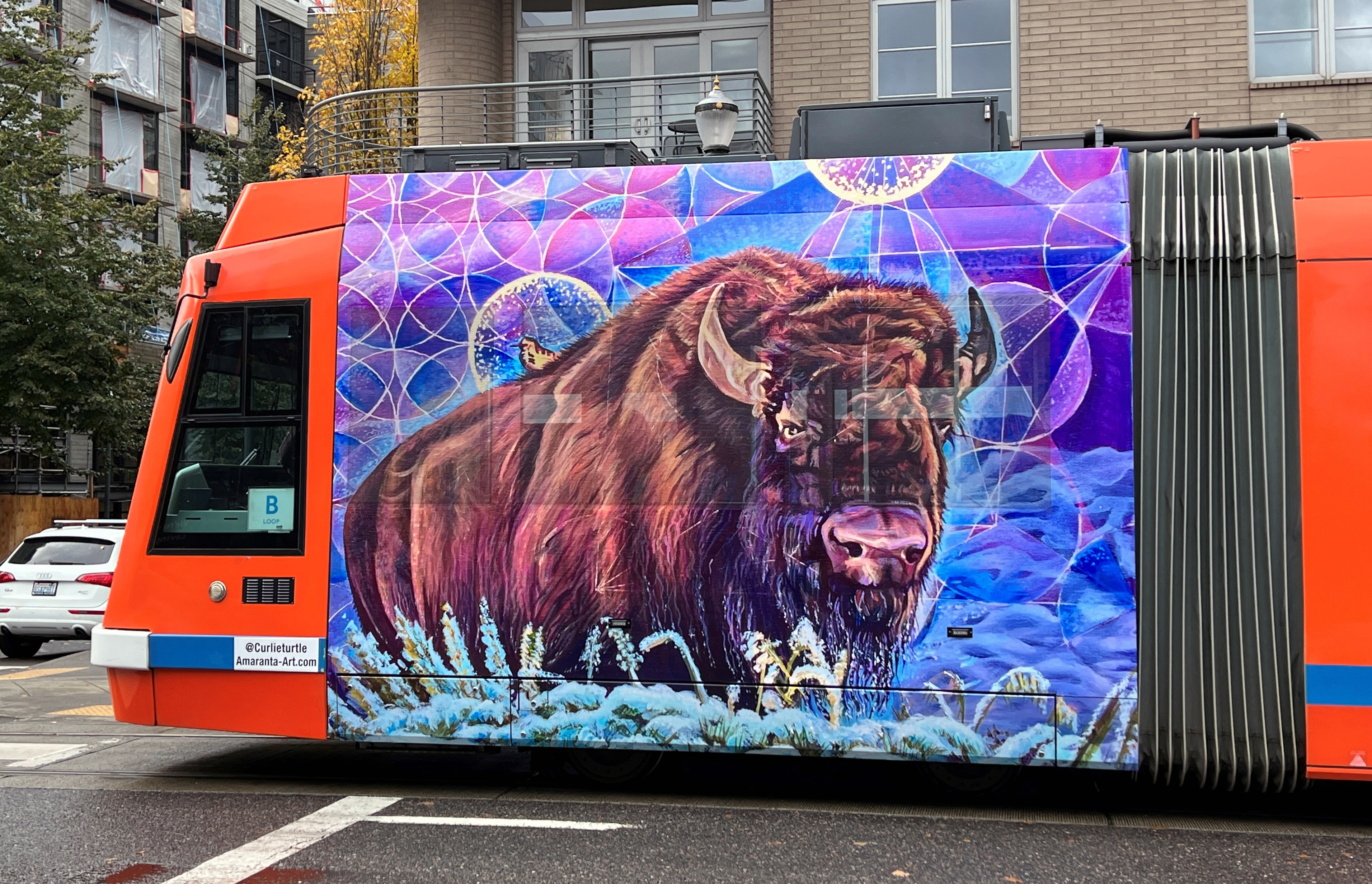The image showcases a bright orange shuttle bus adorned with an intricate mural spanning its entire side. The mural prominently features a majestic brown bison, with rich, traditional brown and darker brown shading, looking directly at the viewer with expressive eyes and a noticeable pink nose. The bison stands in a field of soft, fluffy blue flowers, surrounded by green leaves. Perched on its back is a small, yellow bird. The background of the artwork is vibrant, filled with geometric circles in hues of blue, pink, and purple, resembling a disco ball's reflection. The bus is parked on a street, with a set of apartment buildings visible in the background, adding an urban contrast to the rustic imagery of the mural.